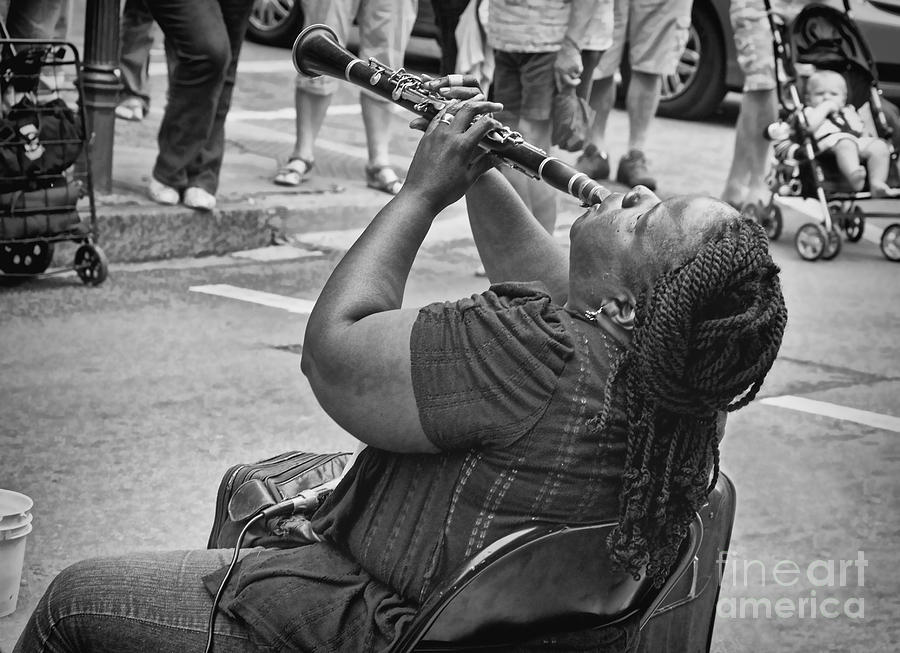This black-and-white photograph, approximately six inches wide by four inches high, taken outdoors during the daytime in a street or courtyard setting, features a woman of African descent sitting in a black metal folding chair. She has rope-style braids that are pulled back from her forehead and cascading down her back. The woman is dressed in a short-sleeve blouse and blue jeans. With her head tilted back and her clarinet raised towards the sky, she appears to be fully immersed in her music. A microphone rests across her lap, and a white bucket is situated nearby on the ground. Surrounding the main subject, an array of people can be seen, many just visible by their legs, with some watching the performance including a baby in a stroller. To enhance the artistic appeal, the image bears the text "Fine Art America" in light gray print in the bottom right-hand corner, with "Fine" in thin lettering, "Art" in a larger font, and "America" below it.